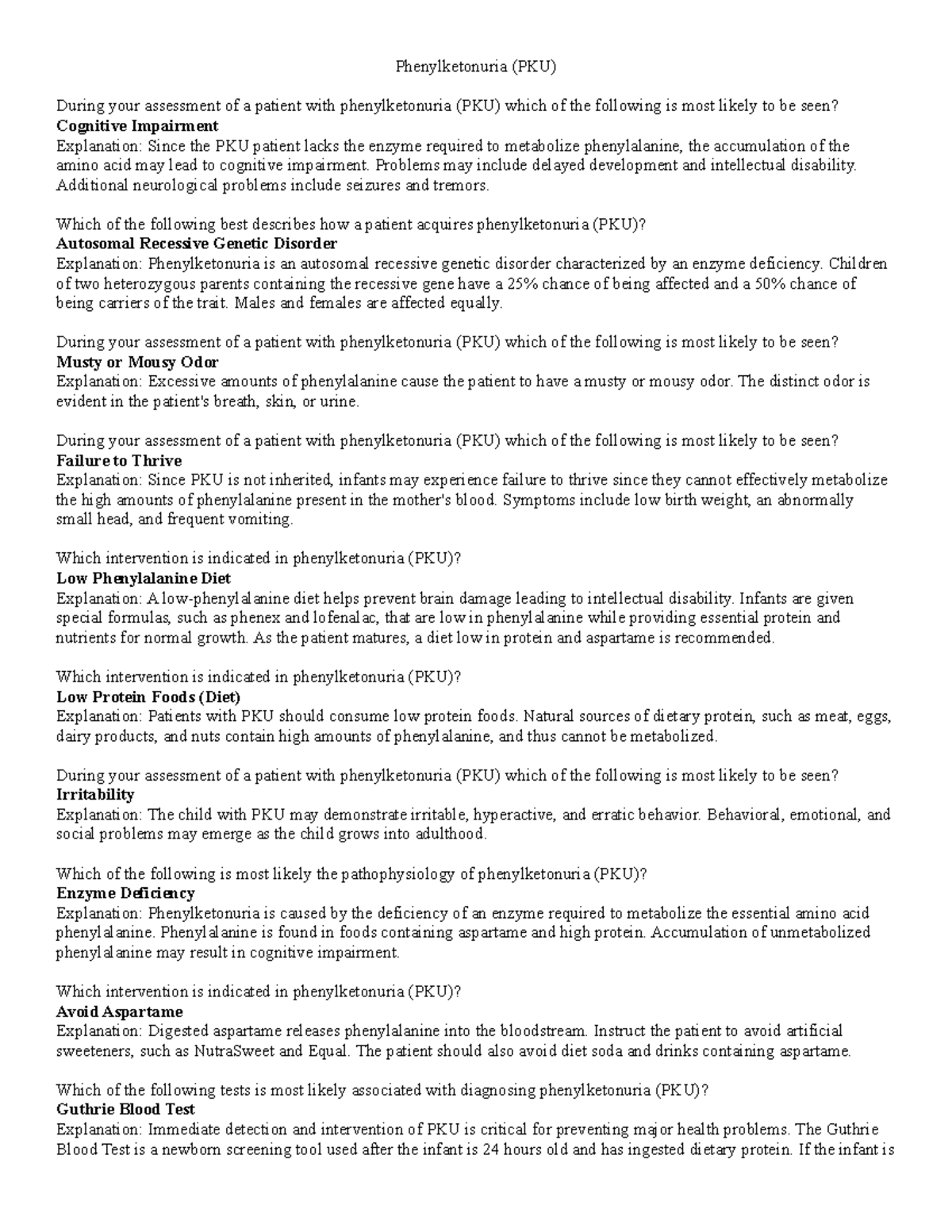The image features a white background with black text divided into ten paragraphs. The title, centered at the top, is "Phenylketonuria (PKU)" with "PKU" highlighted in large letters within parentheses. 

The first paragraph discusses the assessment of a patient with PKU and indicates that cognitive impairment is a symptom commonly seen in affected individuals. 

The second paragraph explains that PKU is an autosomal recessive genetic disorder. 

The third paragraph mentions that individuals with PKU often emit a musty or mousy odor. 

The fourth paragraph notes that failure to thrive is a common condition associated with PKU. 

The fifth paragraph emphasizes the importance of a low phenylalanine diet for managing the disorder. 

The sixth paragraph recommends a diet consisting of low-protein foods. 

The seventh paragraph highlights that irritability is another symptom linked to PKU. 

The eighth paragraph discusses enzyme deficiency related to the disorder. 

The ninth paragraph advises avoiding aspartame in the diet of individuals with PKU. 

The tenth and final paragraph describes the Guthrie blood test, a diagnostic tool for PKU.